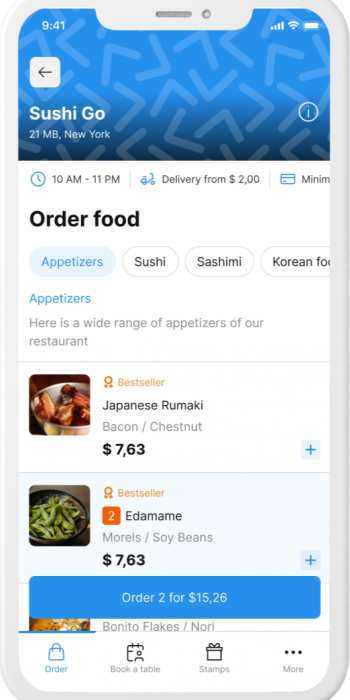The image is a detailed screenshot from a mobile application, presumably for ordering food from a restaurant named "Sushi Go." The top section features a blue background adorned with small triangle patterns, with the restaurant's name displayed in white text at the bottom left corner. The middle section features a white background with key information: operating hours from 10 a.m. to 11 p.m., a delivery fee starting at $2, and an option to "Order Food" in bold black lettering.

Below this, users can choose from various categories for their order: Appetizers, Sushi, Sashimi, or Korean Food, with the "Appetizers" category highlighted. A text in blue beneath the appetizers selection reads, "Here is a wide range of appetizers from our restaurant."

The first appetizer, marked as a "Best Seller," features an image of a bowl filled with a brown dish labeled "Japanese Aromaki Bacon Slash Chestnut" priced at $7.63. The second appetizer, also labeled as a "Best Seller" in orange, shows a green vegetable, identified as "Edamame." It includes a description, "Morels / Soybeans," and is similarly priced at $7.63. Additionally, there's a blue button offering a deal: "Order 2 for $15.26."

The bottom of the screen contains several navigational buttons: "Order," "Book a Table," "Settings," and "More," providing further functionality for the app user.